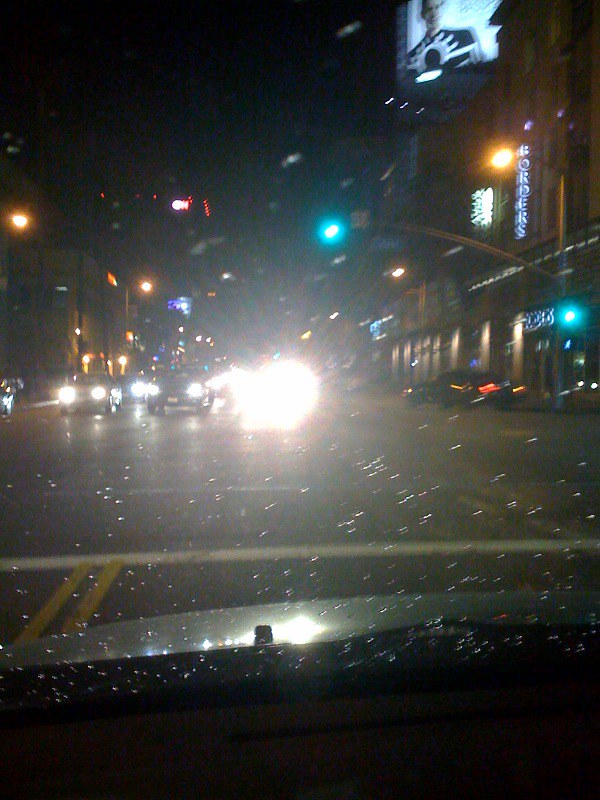The photograph depicts a nighttime urban scene through the blurry windshield of a car, which is speckled with raindrops. The image appears to capture a busy intersection in a downtown city block. Dominating the view is a car directly in front with exceptionally bright headlights, rendering the car itself indistinguishable. Three rows of cars on the left side of the street have their headlights on, contributing to the overall glare. On the right, there is a green traffic light attached to a horizontal pole. 

A car, either parked or moving in the same direction as the vehicle from which the photo is taken, is visible on the right-hand side near the curb. More to the right, the photo showcases buildings adorned with neon lights, including what seems to be a Borders bookstore and a large monitor three stories high displaying an image of a man. The scene is illuminated by various street and building lights, underscoring the urban setting.